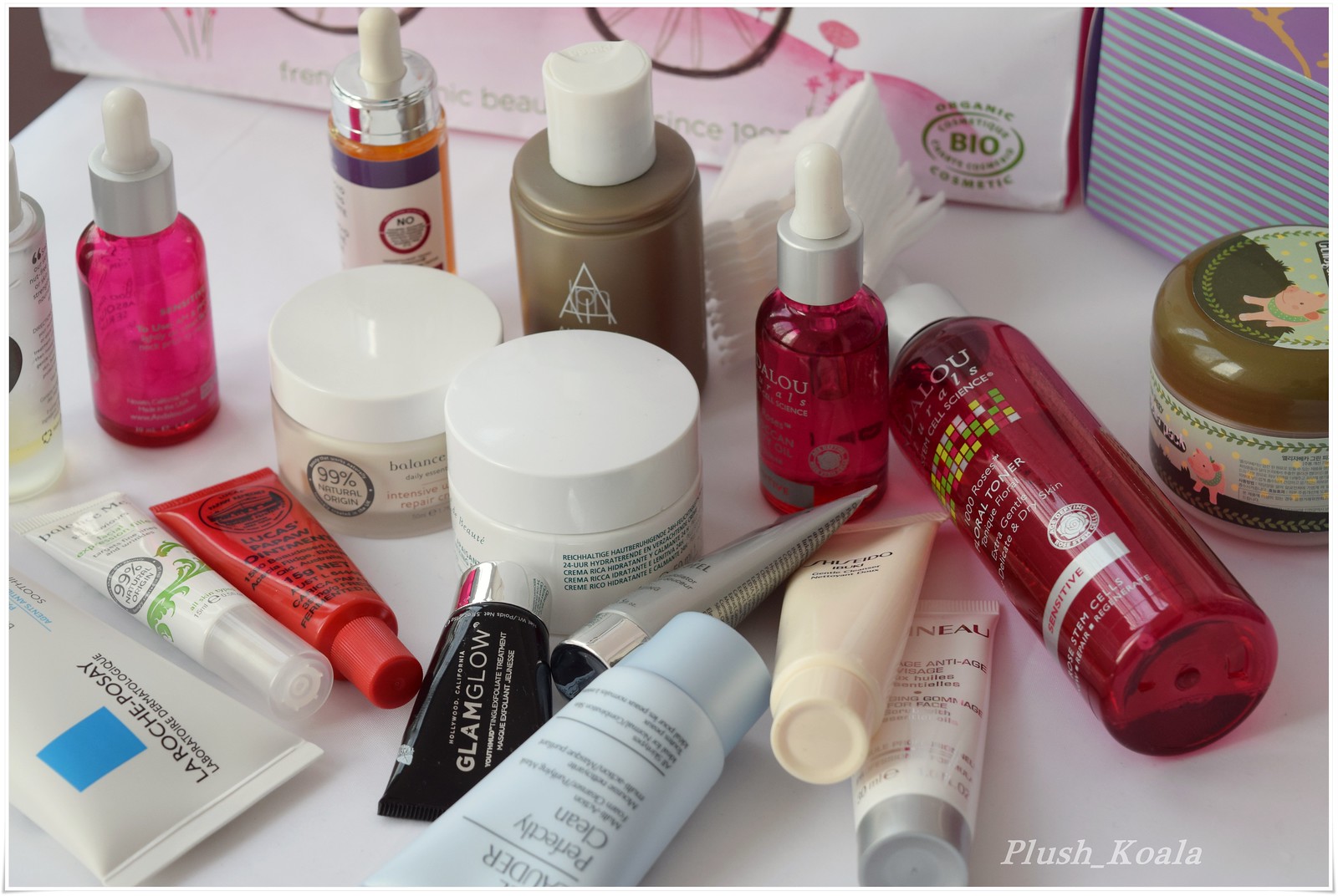An array of cosmetic products is artfully displayed on a pristine white surface. Prominent in the foreground are three elegant bottles with droppers, each a different vibrant hue: one pink, one orange, and one red. Accompanying these bottles are three tubs, presumably containing creams, with one in a rich brown shade and two in clean white. A neat stack of cotton sheets and a container of cotton swabs are positioned towards the back, adding a touch of orderly utility to the scene.

The lower section is populated with various tubes of lotions and creams, meticulously arranged yet enigmatically turned so their labels are not fully visible. A subtle watermark reading "plush_koala" sits unobtrusively in the bottom right corner, marking the image’s origin.

The backdrop contributes to the whimsical atmosphere with a picture of a bicycle perched on a pink hill, evoking a sense of nostalgic charm. To the right, another image with purples and soft blue horizontal stripes adds a modern, abstract touch to the visual narrative. Collectively, these elements combine to create a meticulously composed and visually engaging tableau, where every product and detail invites curiosity and admiration.